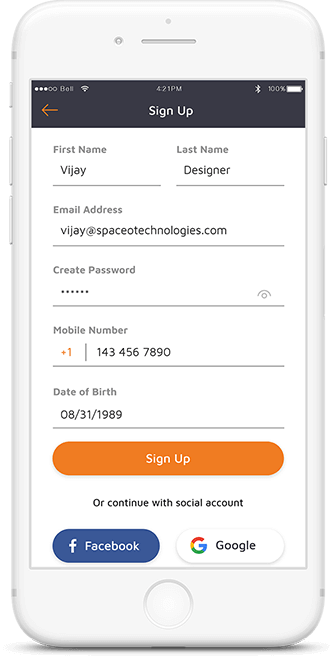A sleek and minimalist white smartphone, which appears to be either an older iPhone or a white Android model, is prominently displayed in the marketing image. The phone features a front-facing camera at the top, and a circular home button at the bottom of its screen. The screen itself showcases a sign-up form for a service.

Displayed on the screen, the form includes fields for:

- First Name: VJ
- Last Name: Designer
- Email Address: vj@spaceotechnologies.com
- Create Password: Represented by six hidden characters
- Phone Number: +1 (143) 456-7890
- Date of Birth: 08-31-1989

Below these fields, there are two prominent options: "Sign Up" and "Continue with Social Account". At the bottom, there are buttons for two social media platforms – Facebook and Google.

The image conveys a clean, modern interface designed to make the sign-up process straightforward and user-friendly.